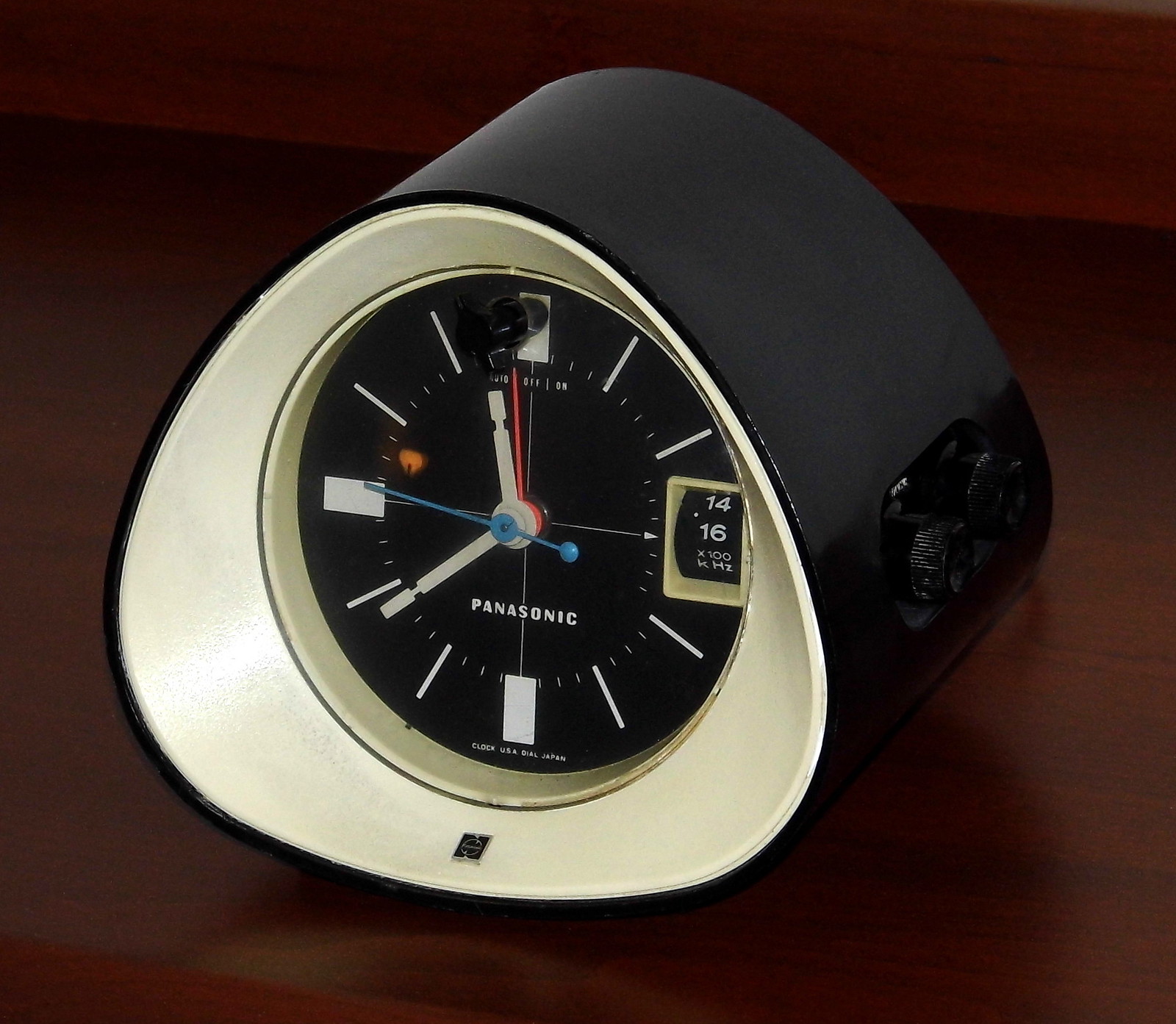The image showcases a unique, vintage bedside alarm clock with a distinctive curved triangular shape and rounded edges. The clock's exterior is black, likely made of plastic, with the brand "Panasonic" inscribed on the front in a simple, retro font. The clock is positioned on a stained wooden surface, which reveals slight color variations in its lines due to the wood grains.

The clock's face features a central white portion with a large black circular dial. The hour and minute hands are white, while the second hand is blue, and there is an additional small red hand indicating the alarm set time. The face is designed with thick white lines at the 12, 6, and 9 o'clock positions but lacks a thick marker at 3 o'clock, which is replaced by a dial displaying "1416" with "X100 KHZ," possibly suggesting an AM radio feature.

The clock's circumference is marked with simplified hour and minute indicators. The top, sides, and front of the clock are visible in the image, showing buttons or settings on the side, hinting at possible functionalities. The clock casts a subtle shadow on the wooden surface, highlighting its three-dimensional form and nostalgic design, reminiscent of the 1960s. The time displayed on the clock is approximately 11:39.